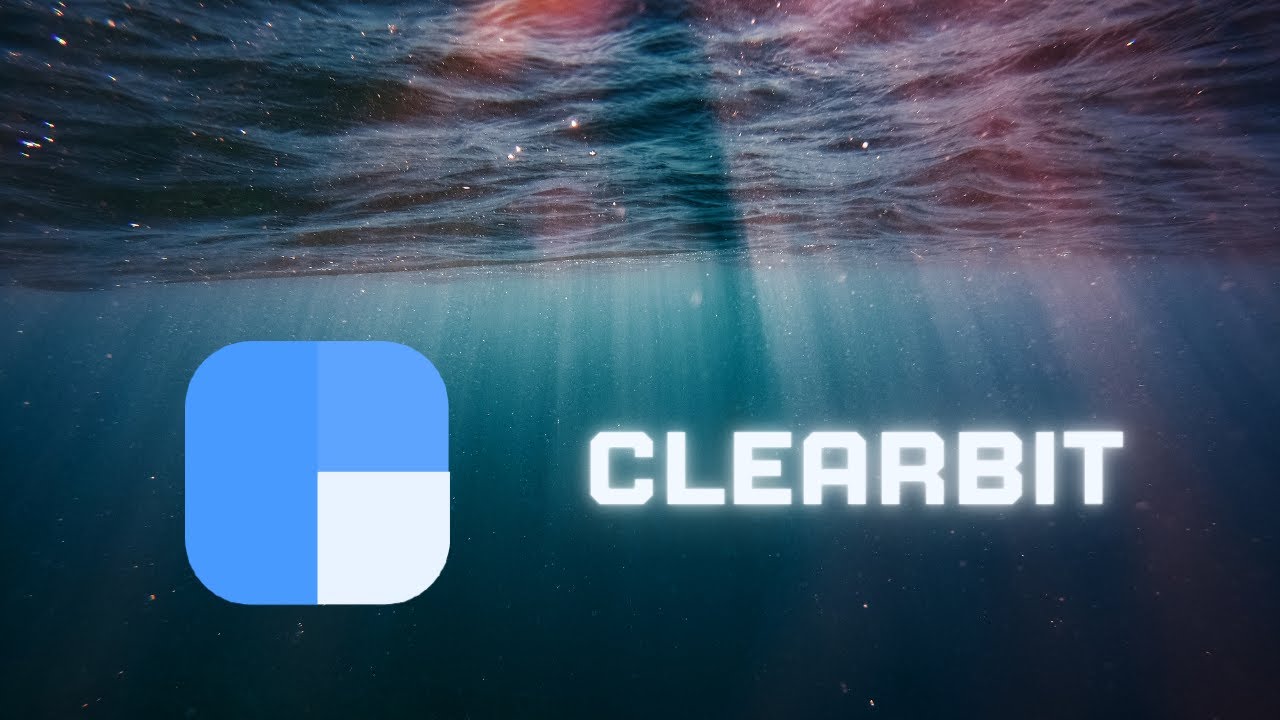The image features the Clear Lit brand logo floating serenely in water. The background is primarily composed of a gradient of dark blue water, lightening as it approaches the surface. The top portion of the image showcases ethereal purple and pink streams of light filtering through and breaking the water's surface, possibly superimposed. The surface of the water is crystal clear, providing a surreal, almost magical ambiance.

Positioned just below the middle of the center and slightly to the right, the "Clear Lit" logo is prominently displayed. The text "CLEAR LIT" is written in slightly illuminated white, all in capital letters, enhancing its visibility. To the left of the text is the brand's iconic logo, a square with rounded corners. The left side of this square is a lighter blue color. The right side is subdivided into two smaller squares: the top section is a muted grayish-blue, and the bottom section is a light whitish-gray.

The overall composition exudes a tranquil, yet vibrant underwater atmosphere, effectively highlighting the Clear Lit branding.